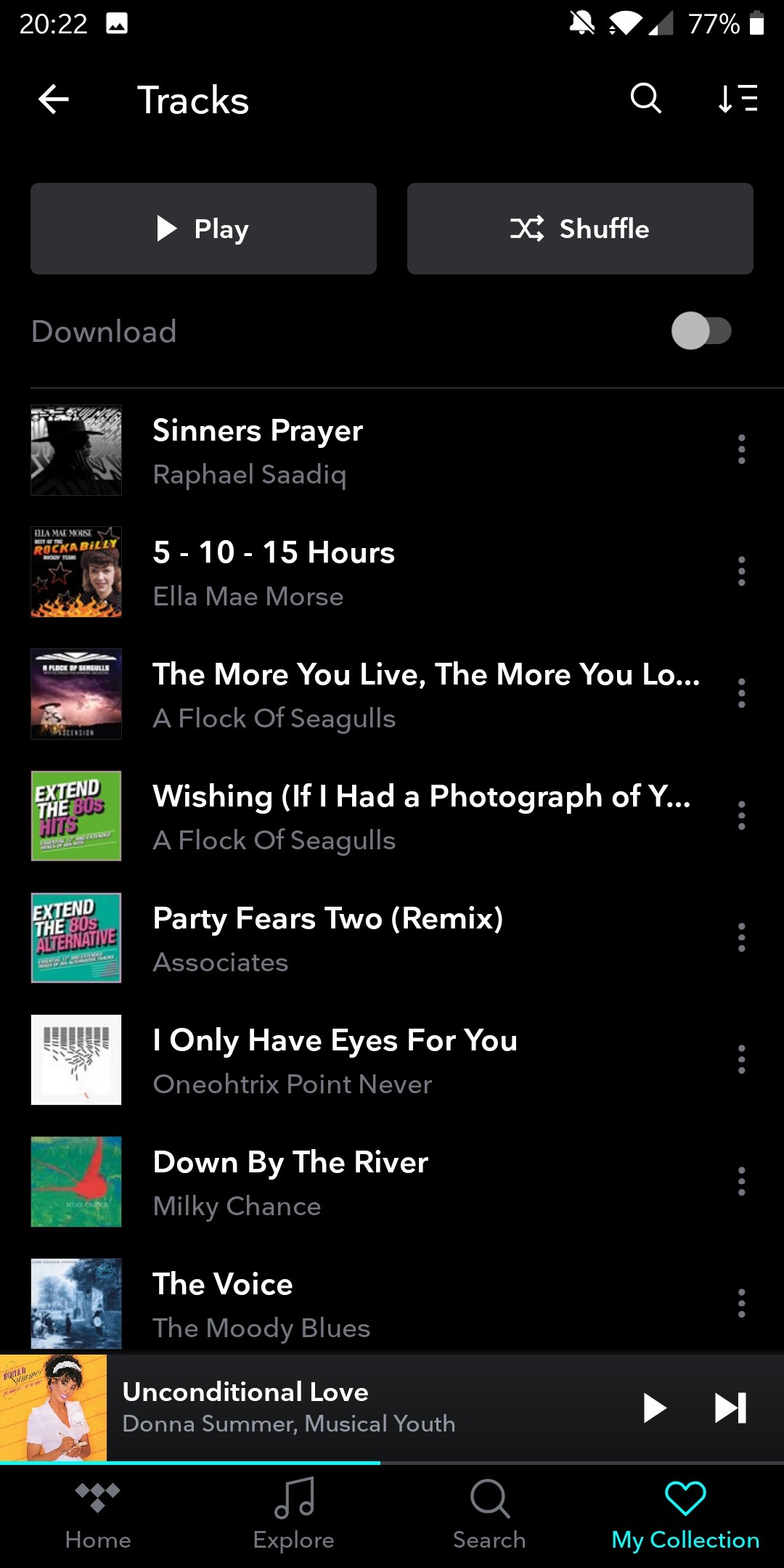The image depicts a music player interface on a cell phone, with the current time displayed in the upper left corner as 20:22. The phone's battery life is at 77%. At the top of the screen, there is a visible left-pointing arrow and next to it, the word "Tracks". Below this, there are control options including a play button represented by a right-pointing arrow and a shuffle option.

The word "Download" appears at the top, followed by a list of songs: 

1. "Sinner's Prayer" by Raphael Saadiq
2. "5-10-15 Hours" by Ella Mae Morse
3. "The More You Live, the More You Love" by A Flock of Seagulls
4. "Wishing (If I Had a Photograph of You)" by A Flock of Seagulls
5. "Party Fears Two (Remix)" by Associates
6. "I Only Have Eyes for You" by Oneohtrix Point Never
7. "Down by the River" by Milky Chance
8. "The Voice" by The Moody Blues
9. "Unconditional Love" by Donna Summer and Musical Youth

The currently playing track is "Unconditional Love" by Donna Summer and Musical Youth. There is a blue progress bar beneath the track, which indicates that the song has been played a little less than halfway.